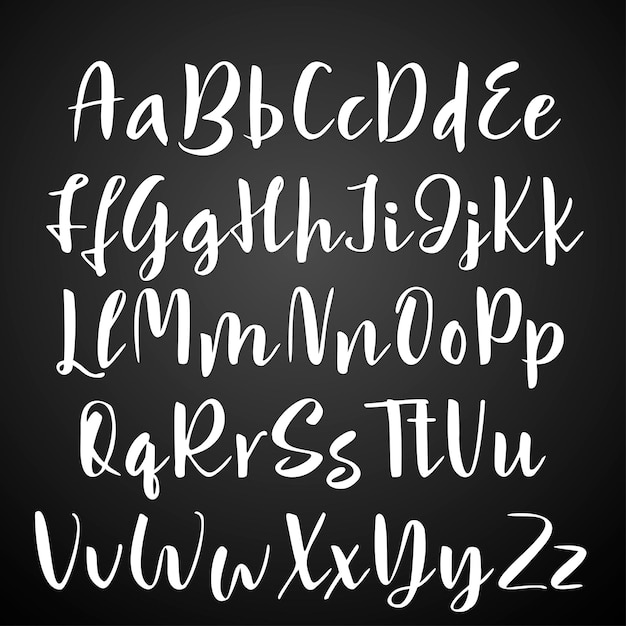The image depicts the full English alphabet elegantly written in white cursive letters on a dark gradient background. The edge of the background is almost black, gradually transitioning to a lighter shade towards the center, creating a subtle gradient effect behind the central portion of the letters. Each letter of the alphabet appears twice, with the uppercase letter followed by its lowercase counterpart, arranged sequentially from A to Z (A, a, B, b, C, c, D, d, and so on). The cursive script is wide and flowing, providing a classic and sophisticated appearance to the alphabet in this detailed and visually captivating presentation.